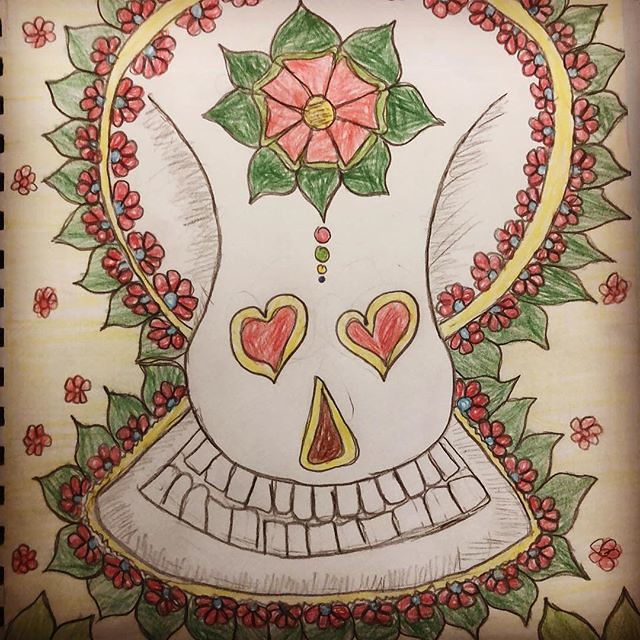This intricate colored pencil drawing on plain white paper features an artistic hybrid of a skull and a vase. The central figure appears vase-like, with the rounded upper part resembling a bulbous, non-traditional skull, and a flared base forming a wide, toothy grin. The eyes are depicted as vibrant red hearts with yellow borders, adding a whimsical touch. Below the eyes is a nose shaped like a triangular Hershey kiss, colored brown with a yellow border. Crowning the top of the skull-vase is a striking red multi-petaled flower, possibly a lotus, with a yellow center and green leaves, reminiscent of a cartoon sun. Surrounding this main floral element are numerous smaller red flowers, green leaves, and what appear to be tiny red pomegranate seeds, all contributing to the lush, flowery aesthetic. The entire composition is highlighted by a golden halo, enhancing its artistic and otherworldly appeal.